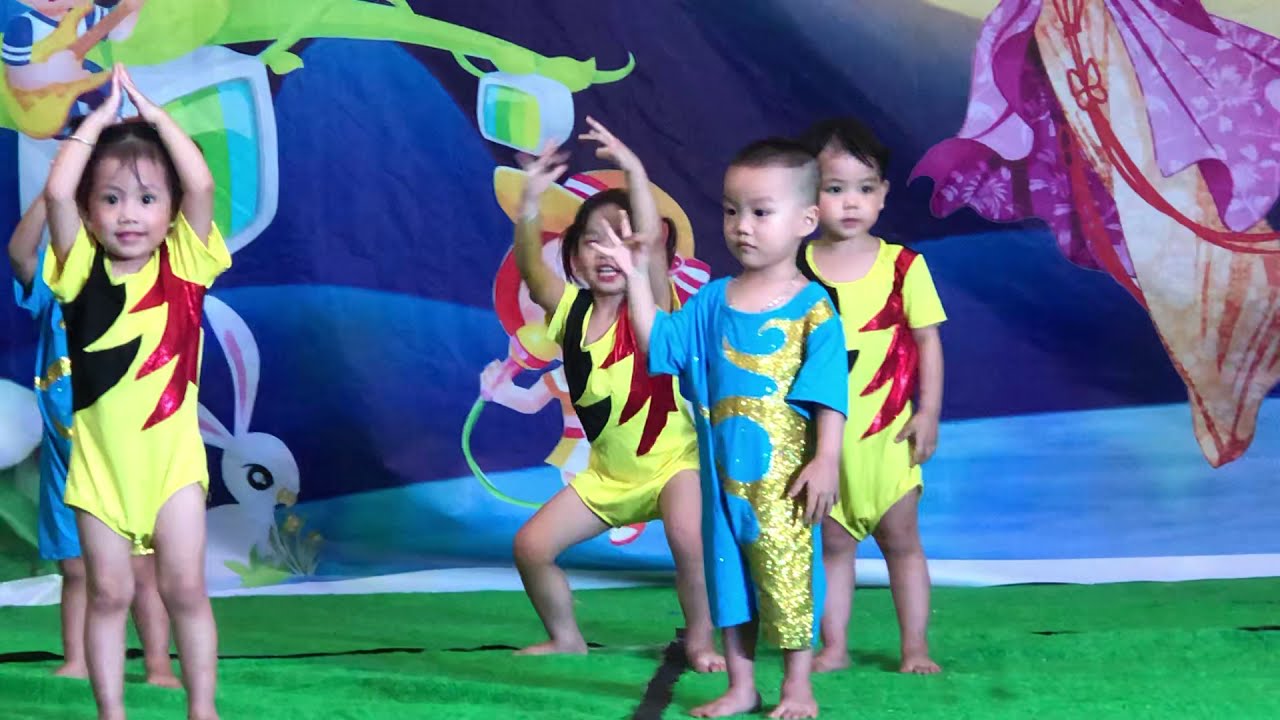The image features five young Asian children, likely toddlers, engaged in a performance on stage. The children are dressed in vibrant costumes: three girls are clad in neon yellow onesies with red and black zigzag stripes, while two boys wear light blue onesies adorned with shiny gold flame designs. All of the children have black hair. The stage is set against a beautifully decorated oriental-style backdrop featuring intricate designs in blues, purples, maroons, and greens, with a notable white rabbit illustration. The floor is covered in artificial green fabric that resembles grass, and the scene is well-lit, highlighting both the colorful setting and the children's expressions, which range from happy to a bit nervous.